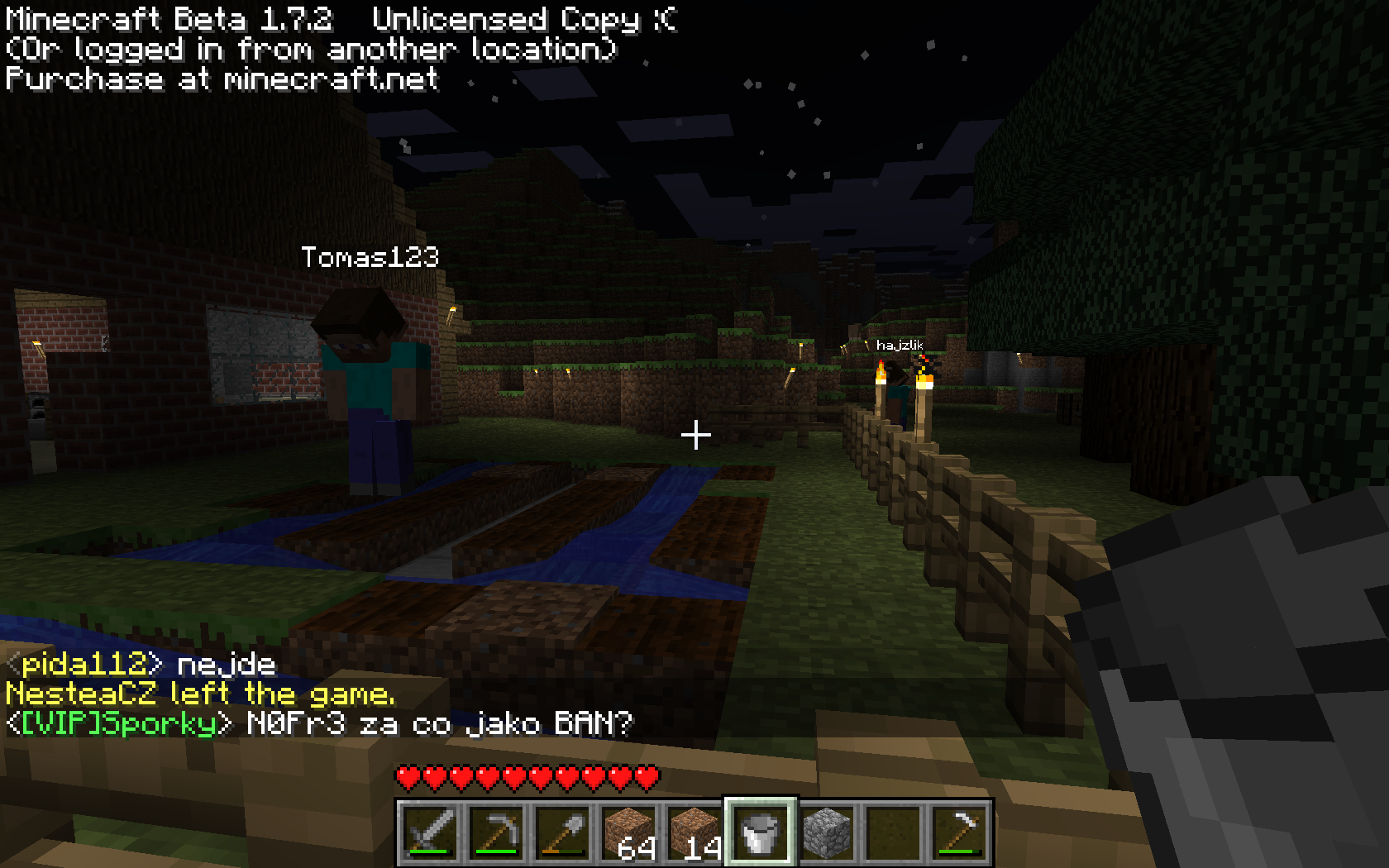The image captures a nighttime scene from the game Minecraft, specifically a screenshot from the "Minecraft Beta 1.7.2, Unlicensed Copy" version, as indicated by the white text at the top of the screen. The landscape is cloaked in darkness, with shadows enveloping most of the elements within the frame.

On the right side of the image, a wooden fence runs parallel to the edge of the scene. Near the center, slightly left, stands a character identified by the overlay text at the top, "Thomas123." This character has dark hair and is clad in blue pants and an aqua shirt, appearing to be gazing downward towards the "camera." The character stands near what seems to be a small pond, reflecting the inky night sky. To the left of the character, a building structure can be seen, adding to the sparse nocturnal landscape. The overall scene exudes a quiet, shadowy ambience typical of Minecraft's night-time environment.